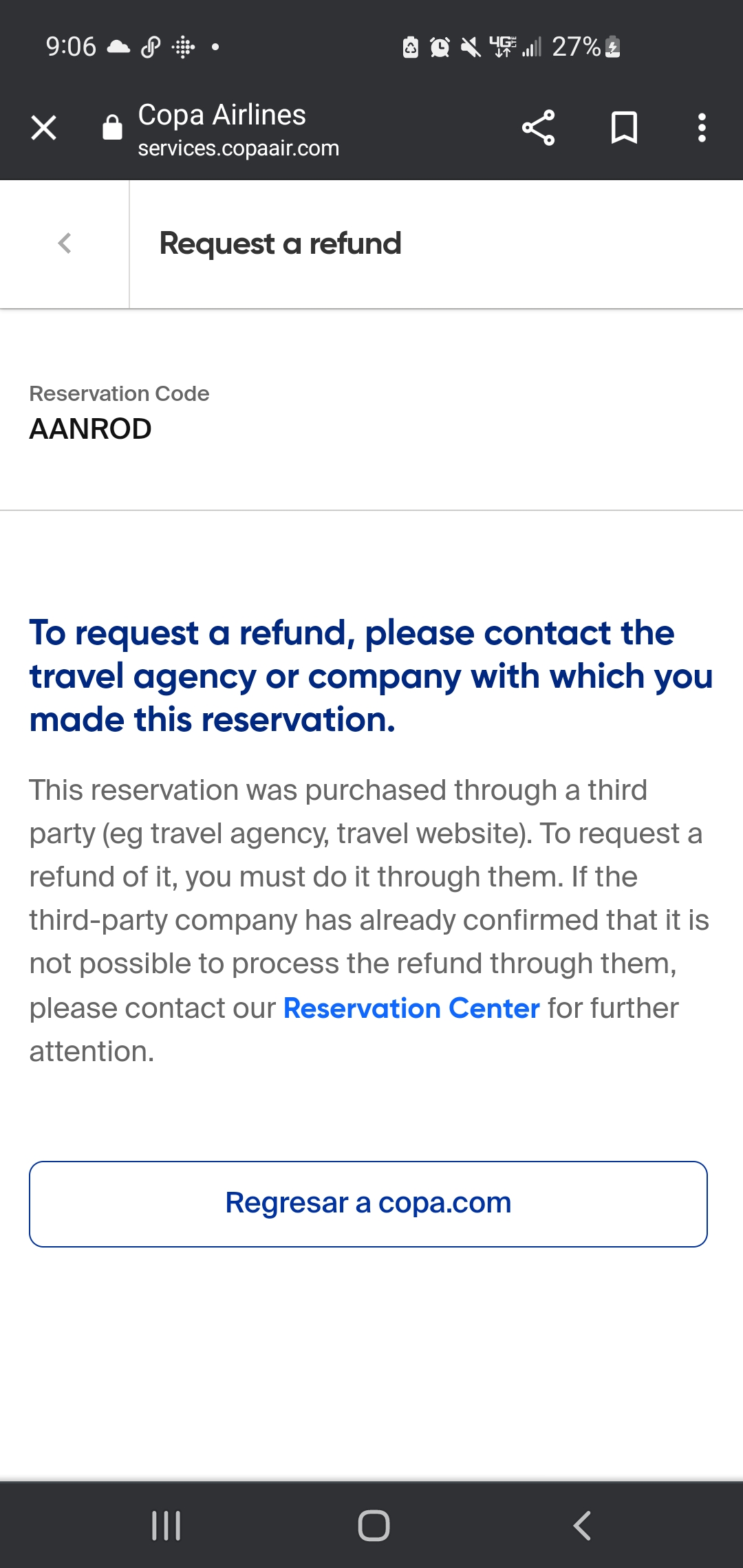This screenshot, apparently captured from a phone, omits external phone borders, showing only the screen's content. At the top, a black status bar displays various icons: a cloud insignia, a link icon, a square turned sideways with small squares inside, a dot, and the battery icon indicating 27% charge. The banner also shows the time as 9:06, along with icons for the clock, volume, 4G signal strength, and battery status.

Below this status bar, on the top left, there is an 'X' icon and a lock icon. The text "Copa Airlines" is visible, followed by the URL "ServicesCopayer.com." On the right side, there are share, bookmark, and three-dot menu icons.

The main content is divided clearly with a line separator. On the left, there is a left arrow icon and the text "Request a Refund." To the right, in bold, is "Reservation Code AANROD," also followed by a separating line. Under it, the instruction "Please contact the travel agency or company with which you made this reservation" appears, highlighted in bold blue.

A detailed body paragraph follows, mentioning a "reservation center" highlighted in blue. At the bottom, a button labeled "Regresar a copa.com" is present.